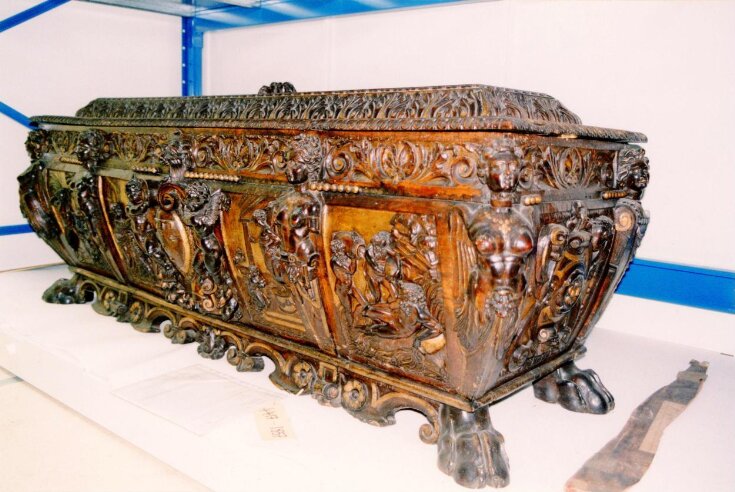The image showcases an ancient wooden casket or coffin, likely displayed in a museum within a protective glass case. The piece is exquisitely and ornately carved, featuring intricate designs that include multiple scenes etched into its sides—four or five on the visible side and another on the end. The carvings include miniature faces and bare-breasted women, giving it a very old-style prestigious design. The wood is predominantly brown with golden and dark green tones, and the lid appears to be designed to open. The casket has feet on each corner resembling hooves or animal feet. Above the scene carvings, small metal tacks or decorations are visible. The surrounding scene includes a white floor, blue baseboards, and a white wall, setting off the detailed craftsmanship of the antique piece.